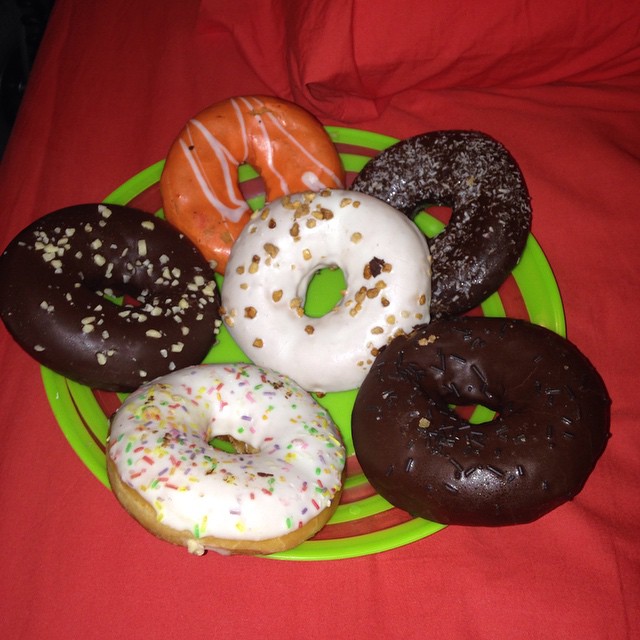The photograph captures a vibrant, crumpled red tablecloth as the background, with a neon lime green plate adorned with concentric red stripes at its center. This dynamic setting highlights six uniquely decorated donuts meticulously arranged in a circular formation on the plate. Each donut brings its own charm:

- At the 12 o'clock position is an orange frosted donut intricately drizzled with white icing.
- Moving clockwise, the 2 o'clock position holds a distinctive chocolate-covered donut sprinkled with coconut flakes or white sprinkles.
- At the 4 o'clock position lies another chocolate-coated donut, this one adorned with chocolate sprinkles.
- Heading towards the 6 o'clock position, a vanilla frosted donut is smothered with vibrant, multicolored sprinkles.
- Positioned at the 8 o'clock mark is yet another chocolate-dipped creation, this time garnished with chopped nuts.
- Rounding it out at 10 o'clock, a chocolate-glazed donut with scattered nuts or coconut pieces catches the eye.

In the center of this delightful circle sits a donut with velvety white frosting, topped with what looks like either burnt coconut flakes or walnut pieces. This photograph, likely taken with flash, showcases the intricate textures and delectable variety of the donuts, presenting a feast for both the eyes and the imagination.